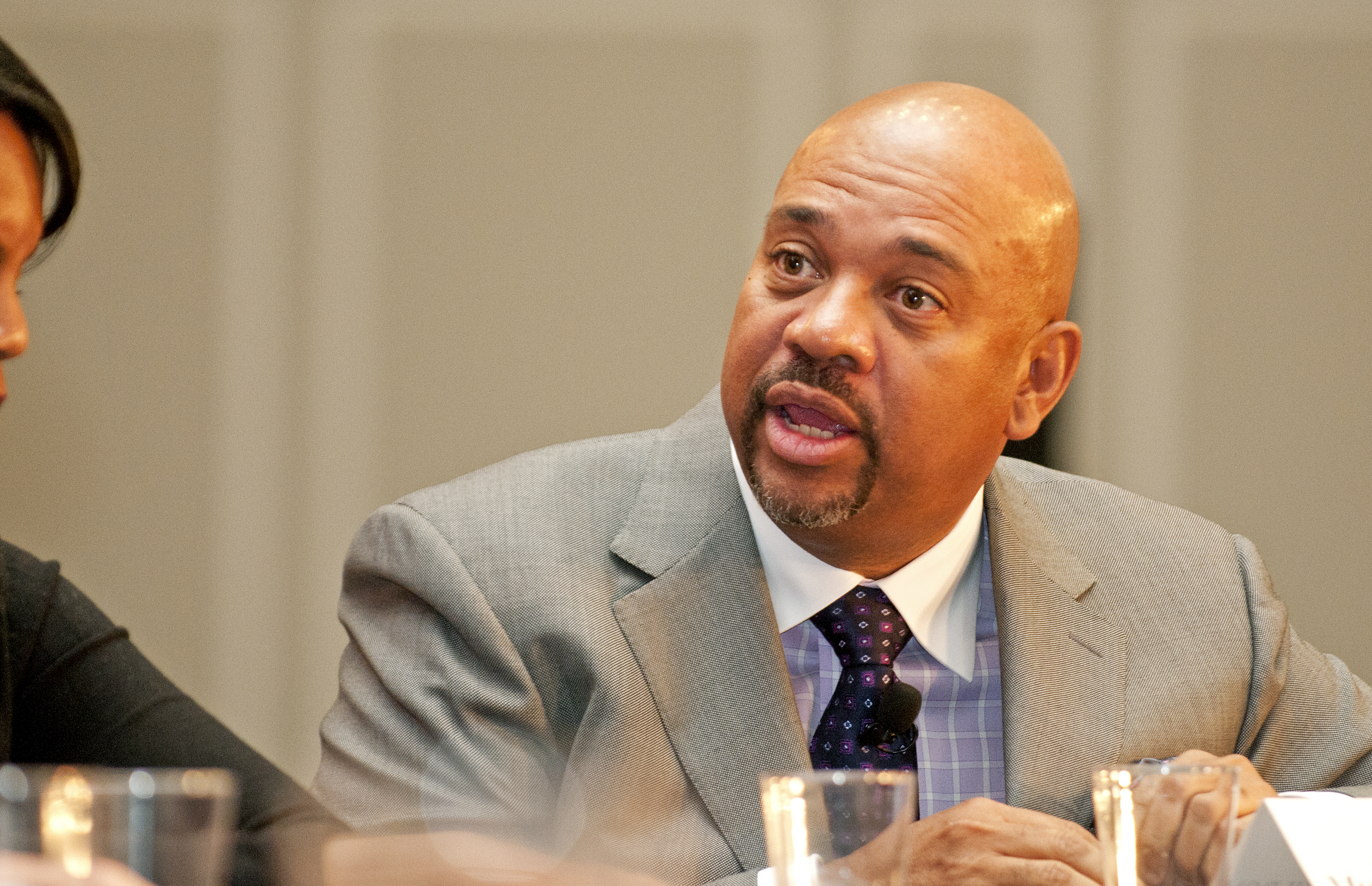This image features Michael Wilbon seated at a table, engaged in conversation with his head turned to the left. He is wearing a light-colored sport coat with a subtle tweed print, a light blue plaid sport shirt with a crisp white collar, and a dark navy necktie adorned with a pink and white pattern. His bald head and dark goatee, graying at the chin, are prominently visible. In front of him, there's a folded name plaque and several clear glasses of water on the table. To his right, barely visible, is a woman with black, side-swept bangs, her profile partially seen including her nose and eyelashes. She is dressed in a dark shirt. The backdrop consists of beige panels or curtains, suggesting an indoor setting that might be an event such as a meeting, debate, or convention. Both individuals have their hands resting on the table, contributing to the formal atmosphere of the scene.